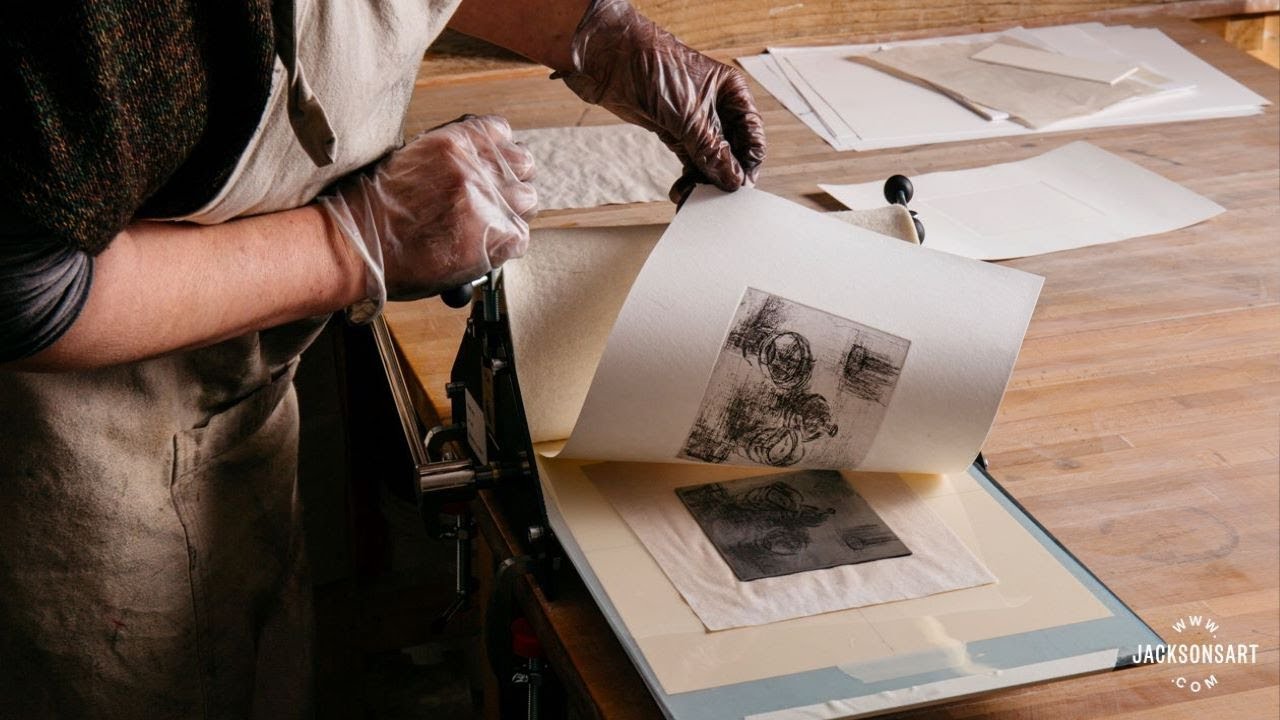The image depicts a person engaged in print work, positioned on the left side of the photo. The individual, whose face is not visible, wears gloves darkened with ink and a canvas apron, suggesting a meticulous and potentially messy process. They are seen peeling a black and white print, possibly from the bottom of a stack of papers, on a wooden table. The workspace is detailed with various sheets of paper, both single and stacked, a possible plastic sheet, and an assortment of tools, encapsulating the art-making environment. The colors present in the image include beige, a brownish leather color, white, and black. The website text "www.jacksonart.com" is found subtly within the image, positioned in the bottom right corner.